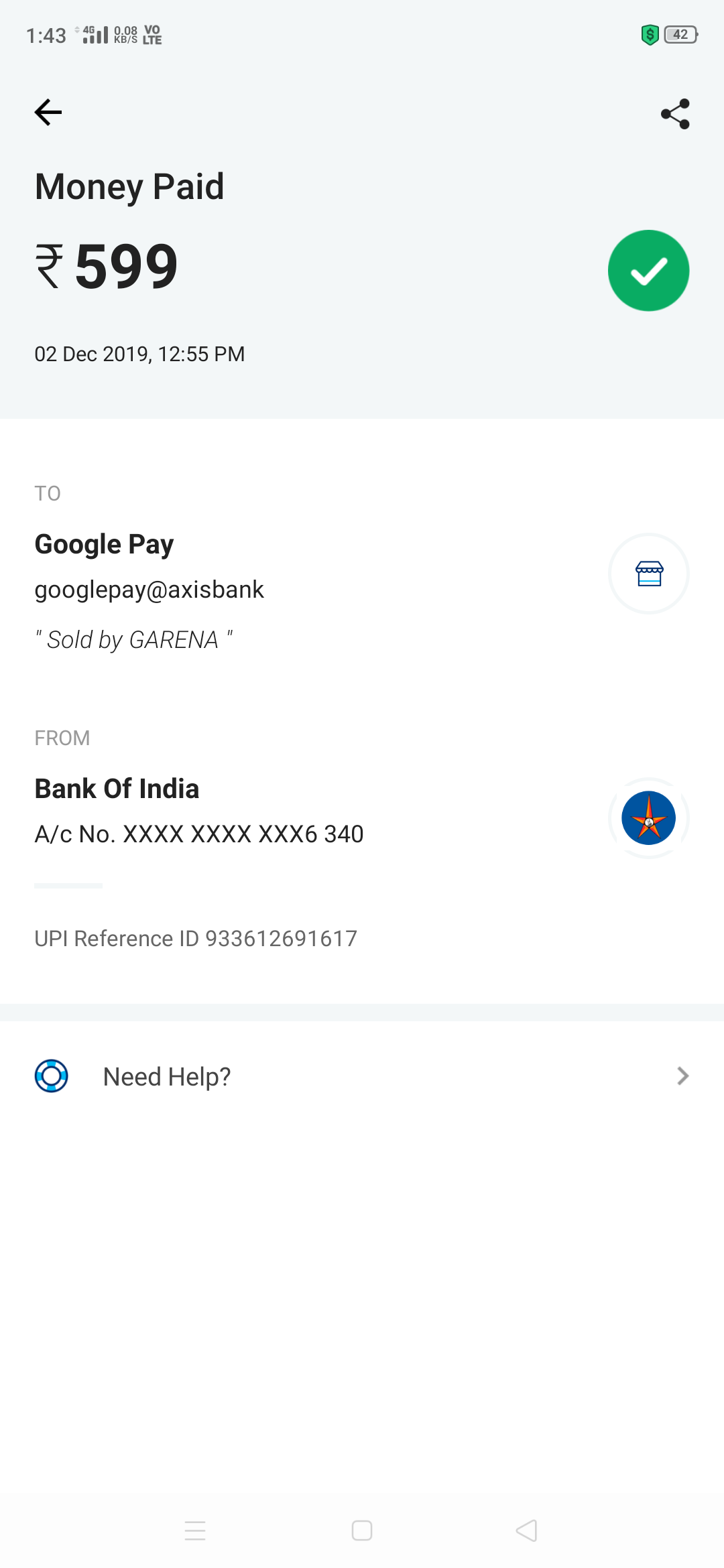The screenshot exhibits a payment confirmation interface with detailed transaction information:

- **Header Section**:
  - At the very top, the device status bar indicates a battery life of 42%, with a 4G connection and full signal bars. The current time displayed is 1:43 PM.
  
- **Transaction Confirmation**:
  - A prominent message at the top reads "Money Paid" followed by the amount, "$5.99". Adjacent to this amount is the symbol for a foreign currency, represented by an "R" with two vertical lines through the circle of the "R".
  - To the right of the amount, there is a green check mark signifying successful payment.
  - Below the confirmation, a share button is available for sharing the transaction details.
  
- **Details Box**:
  - Encased in a light gray box, the detailed transaction information is provided:
    - "02 December 2019 at 12:55" indicating the date and time of the transaction.
    - The transaction was completed via Google Pay at Axis Bank.
    - In smaller, italicized, and gray text, it states "Sold by Garena" to the right, accompanied by an icon resembling a shop with a canopy.
    - Below this, the information "From Bank of India" is bolded.
  
- **Bank Details**:
  - Beneath "Bank of India" is the account number (A/C) displayed as "xxxx-6340," with the last four digits visible for privacy.
  - Adjacent to this is a starfish icon.
  - Below the account number, it mentions the "UPI reference ID," followed by a nine-digit series.
  - At the bottom right, there is a "Need Help" button accompanied by a right-facing arrow.

This meticulous description ensures a thorough understanding of the transactional screenshot, from the interface elements to the specific financial details.